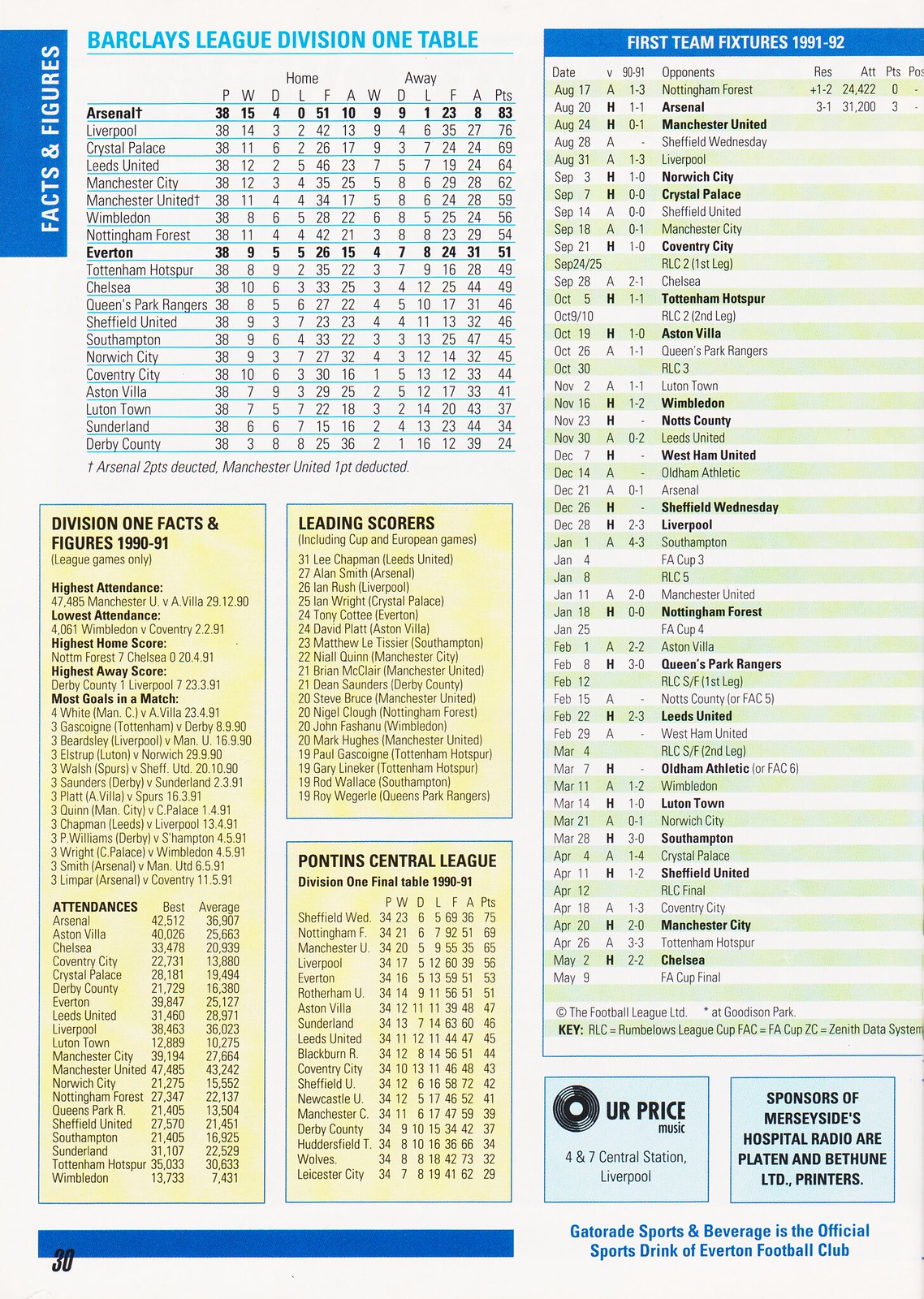This image is from a sports book or program showcasing detailed statistics and standings from the Barclays League Division I for the 1991-1992 season. The main feature at the top is a league table listing various teams, including Arsenal, Liverpool, Crystal Palace, Leeds United, and Manchester United, alongside their home and away game performances and points. Notable dates from August 17th to May 9th are highlighted, tracking the fixtures for these teams. On the left side, yellow boxes present Division I facts and figures, such as highest and lowest attendances, highest home and away scores, and leading scorers. Additionally, there's information about the Pontins Central League Division, with team names and points. Advertisements are placed at the bottom right, including promotions for Gatorade, the official sports drink of Everton Football Club. The page itself is divided into columns with blue and yellow sections, and marked as page 30 in a blue rectangular shape on the lower left. The design incorporates various fonts and colors, such as the sans serif font in blue for certain advertisements.